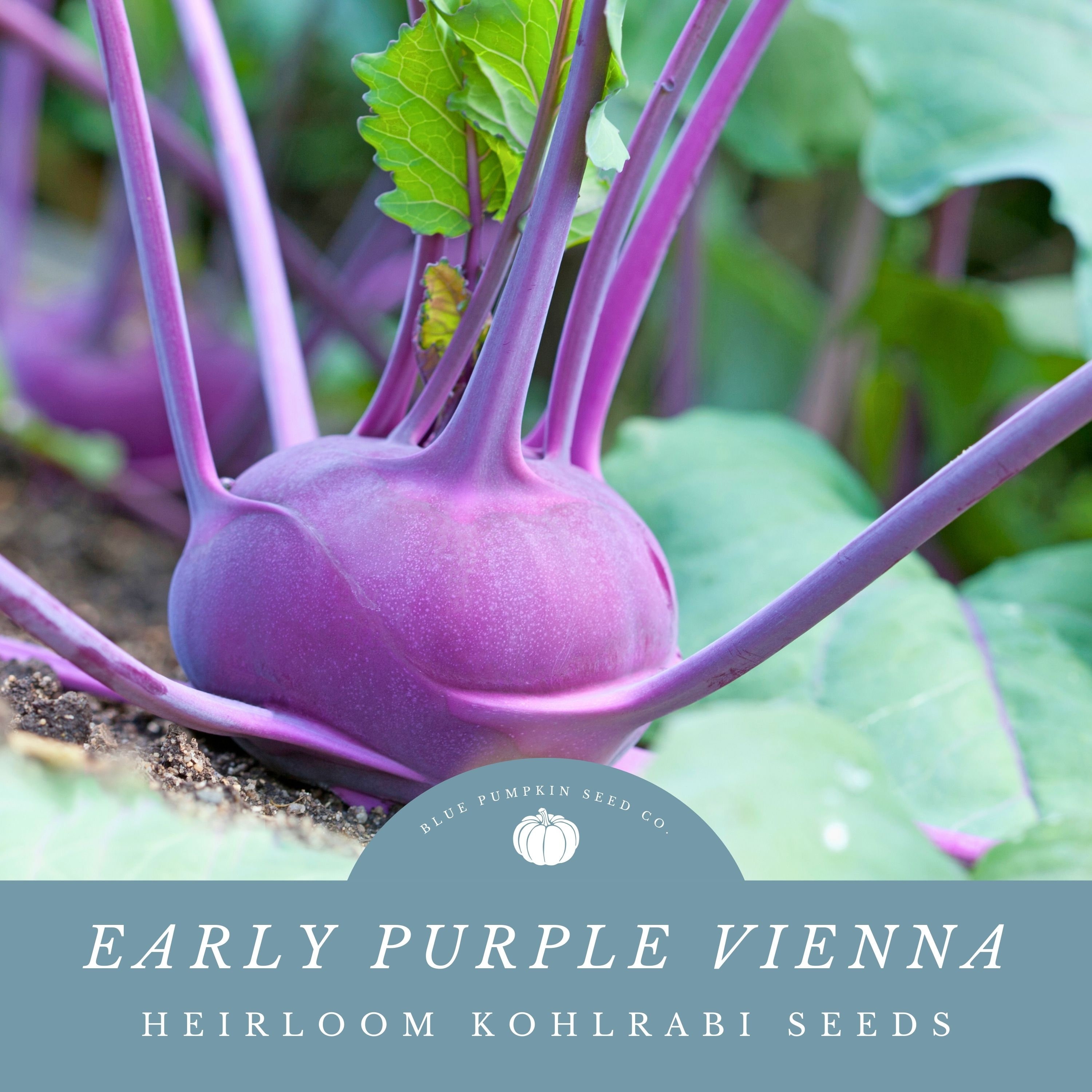The image features a close-up of a vibrant purple kohlrabi plant, showcasing a large, round bulb with purple stems branching out from the top and sides. Green leaves sprout from the stems, while a smaller yellow leaf peeks out from behind. The blurry background reveals more green foliage and additional kohlrabi plants. At the bottom of the image, a gray banner with a semi-circle in the middle displays the text "Blue Pumpkin Seed Co." alongside a white illustration of a pumpkin. Below this, in all capital white letters, are the words "Early Purple Vienna" and "Heirloom Kohlrabi Seeds."